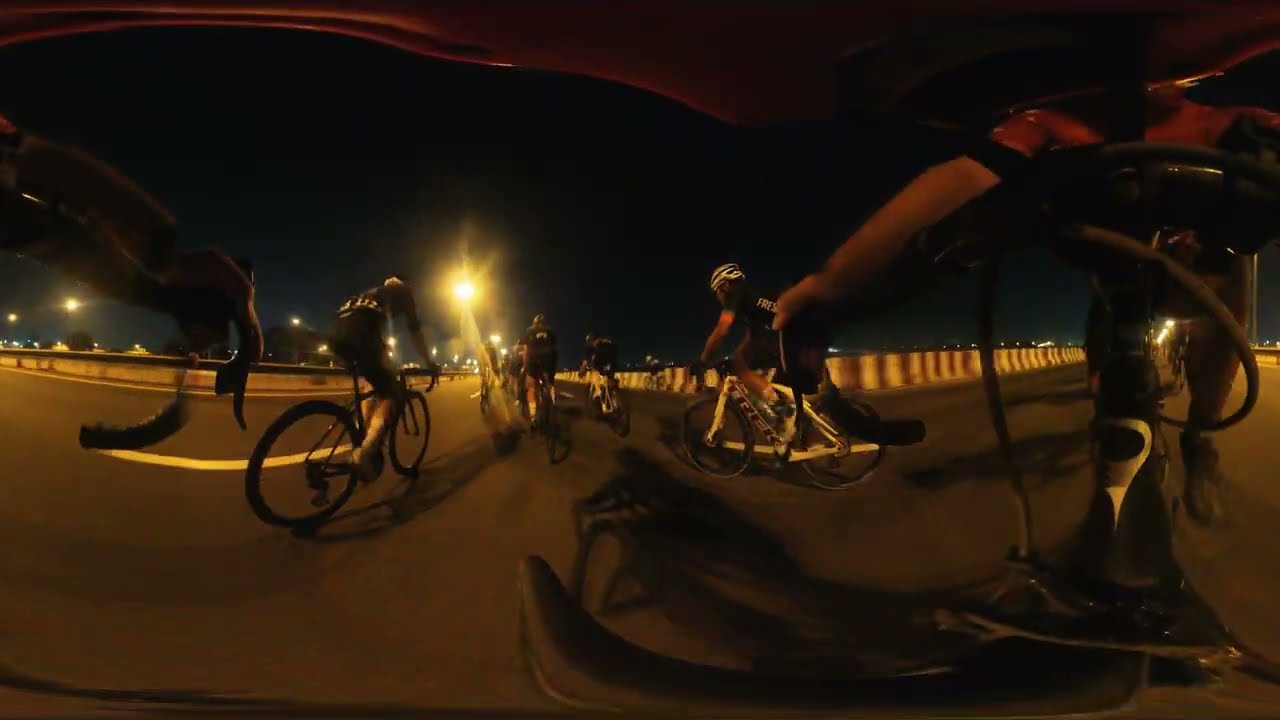The image captures a nighttime scene with a black, almost navy sky illuminated by distant streetlights and devoid of cars. The primary focus is a group of people riding bicycles on an asphalt roadway with white line markings. There are several bikers dressed in tight black and white spandex biking attire and helmets, creating a uniform appearance. The image is heavily distorted with wavy and curvy elements, making it challenging to discern precise details. One rider on the right side appears particularly distorted, only their left arm holding the handlebar is somewhat clear. In the background, a barrier with vertical white and brown stripes is visible, adding to the surreal and almost eerie ambiance. The whole group seems coordinated, possibly participating in a race or a group ride, contributing to a cohesive yet chaotic visual narrative.